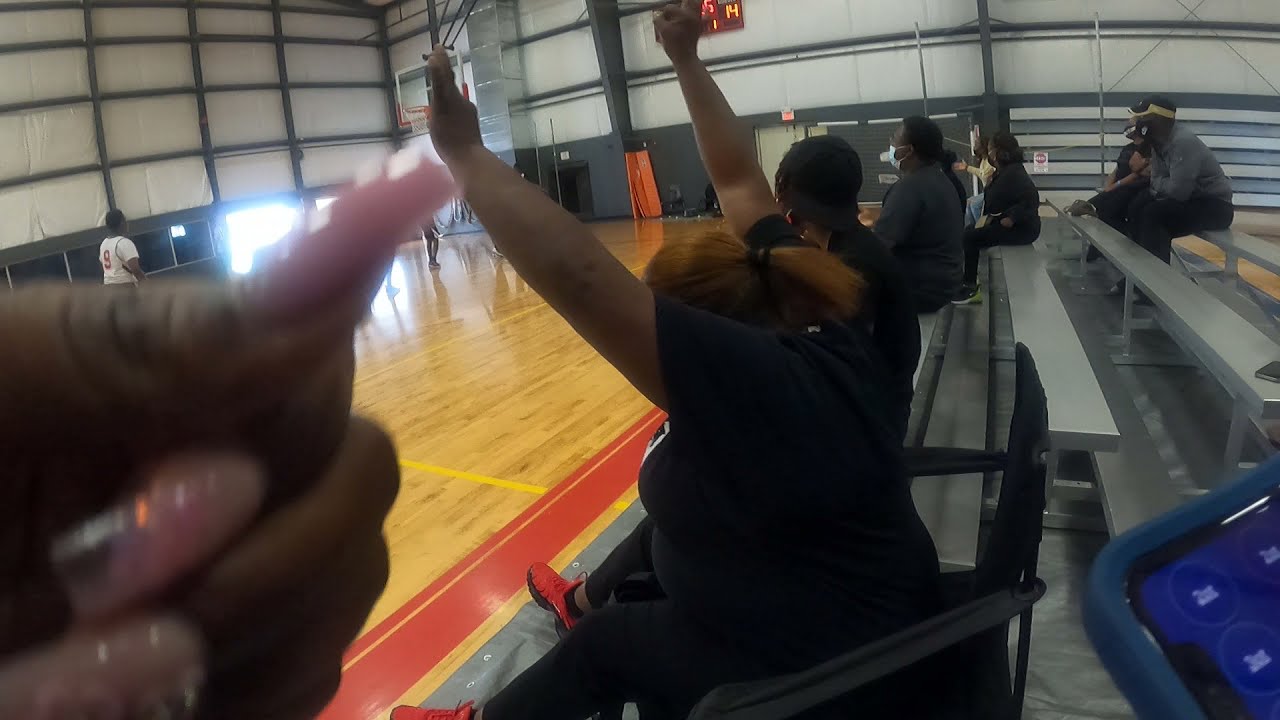The photograph captures a lively scene inside a gymnasium during a youth basketball game. The image is taken from the bleacher section, where around eight spectators, primarily African-American, are seated on silver-gray metal stands, passionately watching the match. In the forefront, a woman dressed in a black t-shirt and black leggings, with red sneakers and red-dyed hair tied back in a short ponytail, is raising her hands in excitement as if cheering for her team. Dominating the left corner of the photo, a black woman's hand with long pink acrylic nails makes a gesture towards the court. The basketball court, visible on the left side, is bordered by red and yellow lines and features one hoop. Some young players, likely elementary or middle schoolers, are seen in action. The gym is surrounded by white and gray walls with some exposed metal and bars, interspersed with canvas-like material, all illuminated by bright fluorescent lights. An electronic scoreboard hangs on one wall, tracking the game's progress.